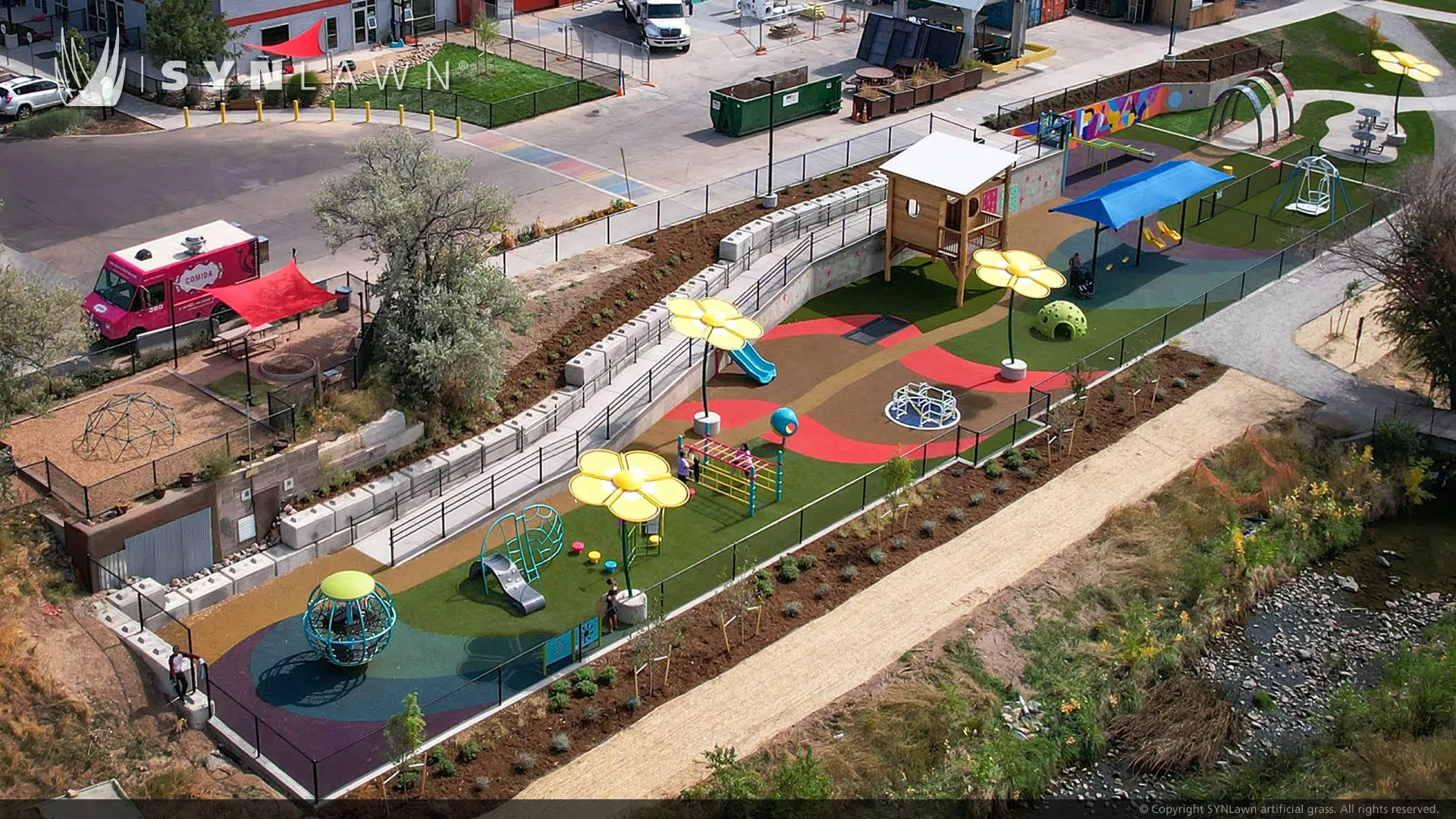The aerial photograph depicts a vibrant and recently installed children's playground, possibly within a schoolyard, nestled near a river or creek. The playground is long and rectangular, stretching diagonally from the lower left-hand corner to the upper right-hand corner of the image. The ground is covered in a colorful array of artificial grass in hues of blue, purple, green, brown, and red, creating distinct pathways and sections throughout the playground.

Scattered across the playground are various play structures, including a small carousel-like ride, monkey bars, a fort-like treehouse with a white roof, and a jungle gym with a silver, wavy slide. Notably, there are shade umbrellas resembling yellow flowers providing cover, and a blue roofed section with swings underneath, featuring both swings for older children and yellow swings for babies.

The playground is bordered by a fence, outside of which small new bushes have been planted. Adjacent to the playground, you can also see a parking area with green dumpsters, several work trucks, and a food truck next to a road. Additionally, there is a noticeable logo, "SYNLAWN," superimposed across the top of the image. The entire scene exudes a playful, child-friendly atmosphere with its bright, engaging colors and varied play equipment.